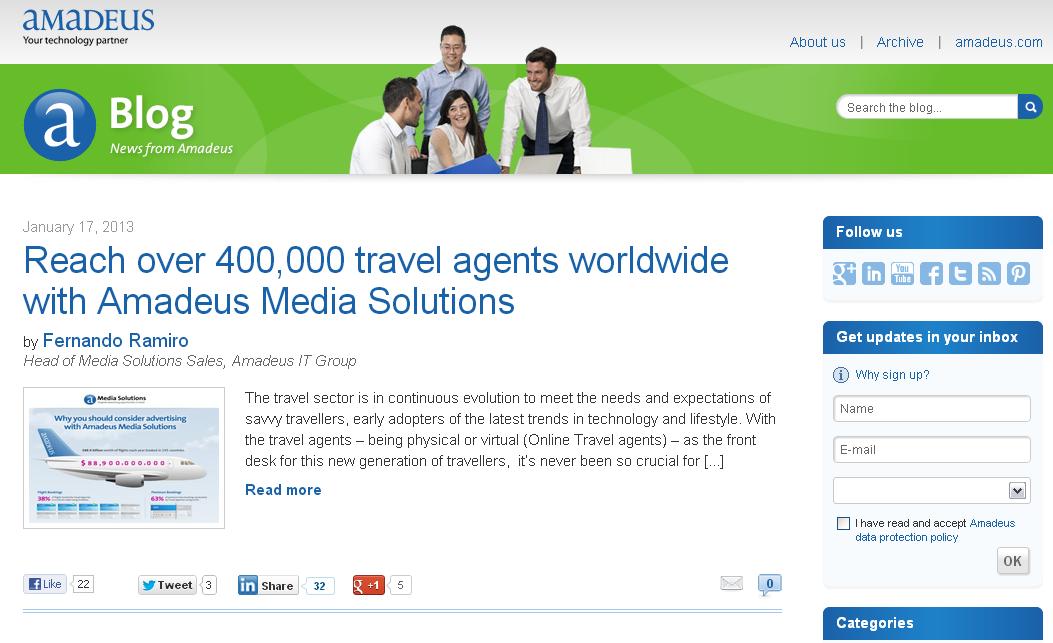The landing page of the Amadeus blog features a prominent top banner. On the left side of this light gray headline banner, the Amadeus brand name is displayed with the tagline "Your Technology Partner" in black text beneath it. To the upper right, there are three navigation links: "About Us" in blue font, followed by "Archive", and "Amadeus.com" separated by vertical lines, directing users back to the homepage.

Directly below, a wide green background banner with light bubble accents in various shades of green spans the page. This banner is adorned with the Amadeus logo—a blue circle with a shiny white bean shape at the top, encasing a lowercase "a". Next to the logo, white text reads "Blog and News from Amadeus."

Centrally located within this green banner are four individuals in business attire—white dress shirts and ties—focused on laptops that face away from the viewer. Two of them are standing, and two are seated, engaging with one another. Among them, one is female and the remaining three are male. On the right side of this banner, there is a "Search This Blog" search bar, featuring placeholder text and a search icon.

The visible part of the blog displays a post from January 17, 2013, with the title "Reach Over 40,000 Travel Agents Worldwide with Amadeus Media Solutions" in blue font. The author, Fernando Ramiro, Head of Media Solutions Sales at Amadeus IT Group, is credited below the title in blue text, accompanied by his title in italicized gray font.

A thumbnail image, resembling an airplane infographic, is situated under the author's name. This image features an airplane flying to the right with pink window details and additional infographic elements below. The post begins with a paragraph describing the evolving travel sector and the critical role of travel agents—both physical and virtual—in catering to the tech-savvy traveler. An ellipsis in square brackets indicates a continuation, leading to a "Read More" button.

To the right of the main content, a "Follow Us" banner in blue lists social media icons for Google Plus, LinkedIn, YouTube, Facebook, Twitter, RSS, and Pinterest in light blue. There's also a "Get updates in your inbox" section with fields for name, email, a dropdown menu, and a checkbox to accept Amadeus's data protection policy, capped by an "Okay" button. Below this is a "Categories" header.

At the bottom of the blog post, users can interact with the content via social media. The post shows engagement statistics: 22 Facebook likes, three Twitter tweets, 32 LinkedIn shares, and five Google Plus +1s.